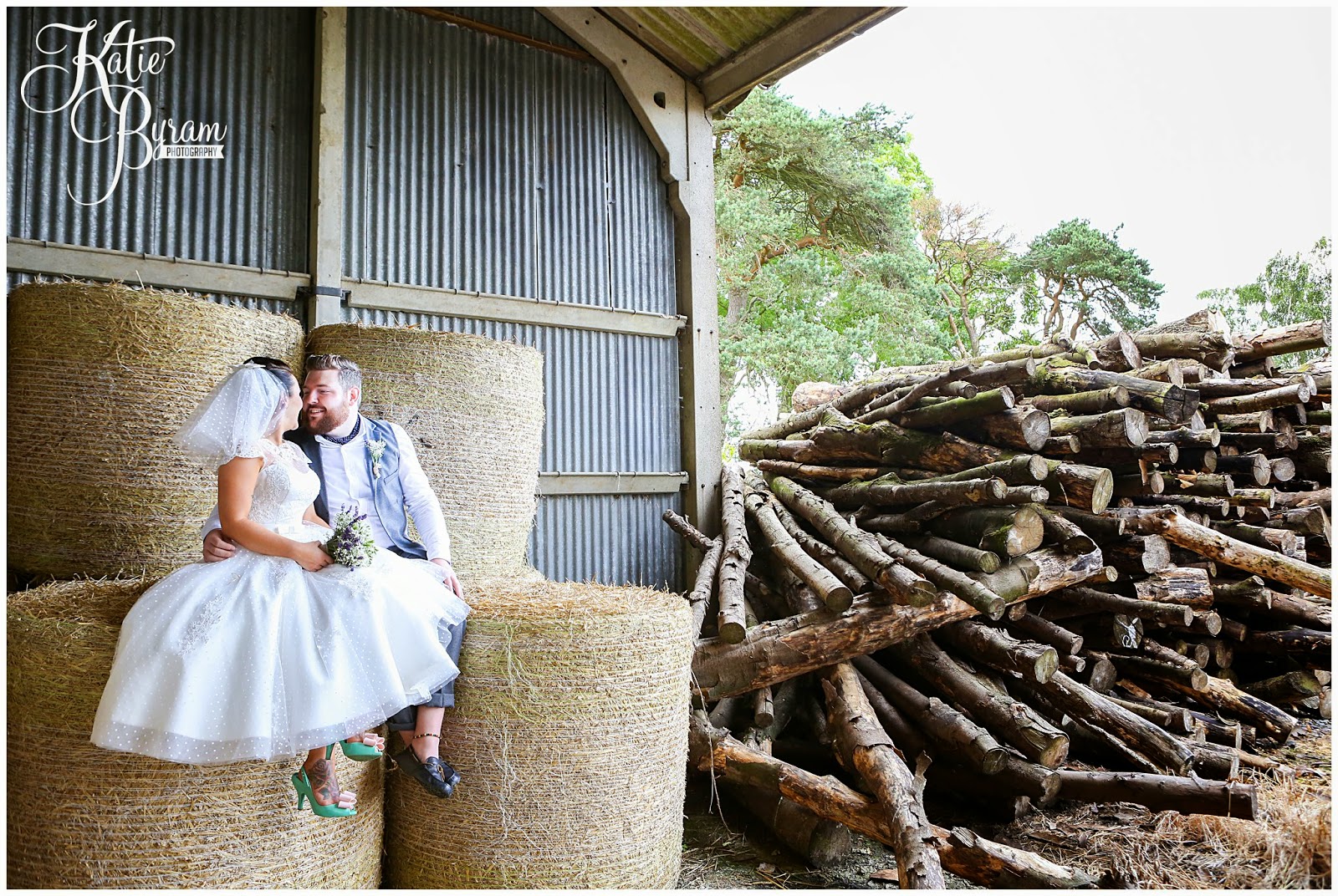The image, showcasing the text "Kate Burnham Photography" in the left-hand corner with large, scripted initials "KB," captures a charming wedding scene set in a barn with corrugated metal and wood framing. The focus is on a bride and groom seated on vertically oriented hay bales, positioned slightly to the left of the center. The bride, adorned in a white wedding dress and holding a bouquet, sports distinct green high-heeled shoes, while the groom, dressed meticulously in a white collared shirt, dark vest, gray pants, and black loafers (without socks), complements her elegance. His groomed beard adds to his polished look. They both share a tender moment, smiling at each other, with her face turned towards him, concealing her features. To the right of the couple, a large stack of cut logs lies on hay-strewn dirt ground, backed by lush green trees. Despite the flat, white appearance of the sky, the setting exudes a bright and serene atmosphere.